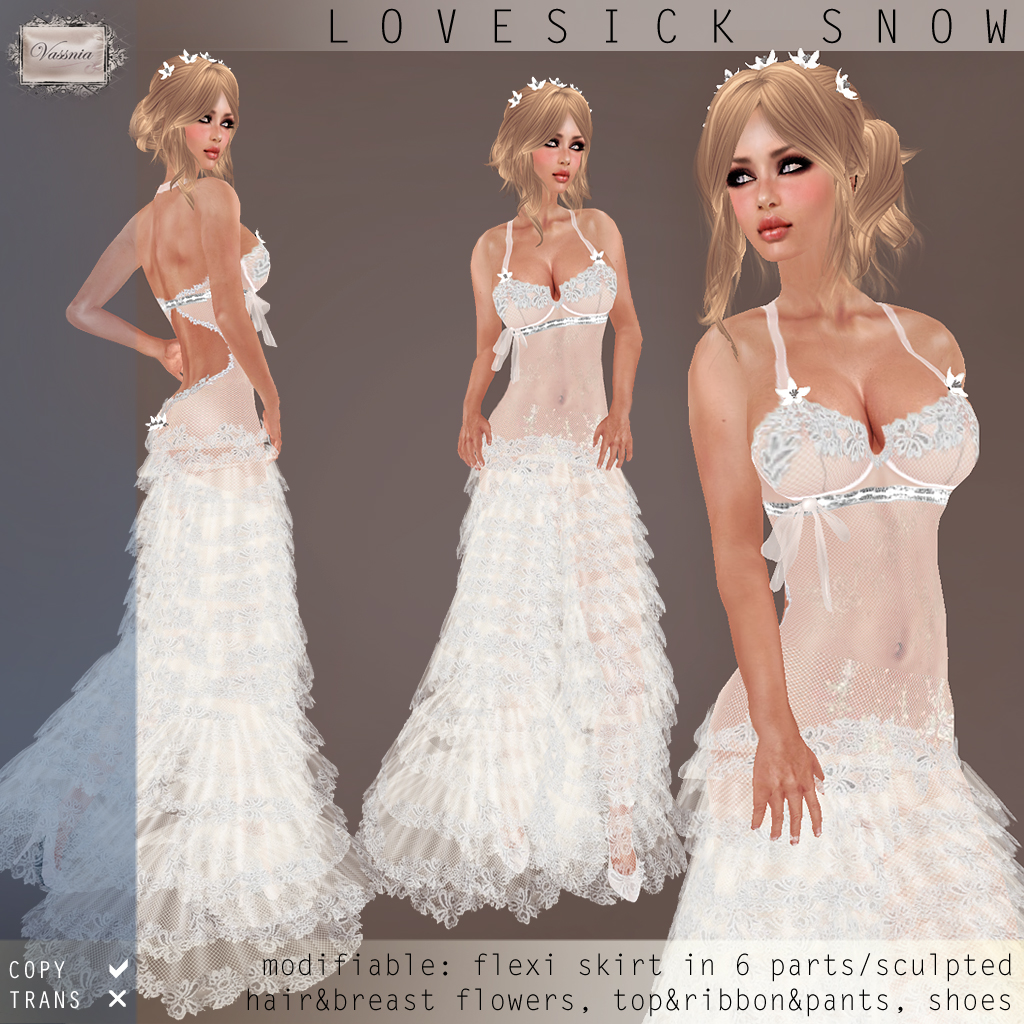This large square image features a dark gray background with a medium gray border at the top, where the words "LOVESICK SNOW" are displayed in all caps black letters. In the upper left-hand corner, there's a logo that reads "VASSINIA." The central area of the image showcases three computer-generated illustrations of a woman, likely the same model, wearing a provocative bridal gown viewed from different angles.

On the left, we see the back and right side of the gown, featuring a bra-like clasp that exposes part of the model's back above and below the clasp, leading down to a ruffled, lacy train. The center illustration shows the front of the gown, highlighting its sheer, see-through lace material over the belly area and delicate spaghetti straps. The gown is form-fitting from the bust to the pubic area, with ruffled tiers extending down to the ground. On the right, a close-up view focuses on the upper portion of the dress, emphasizing its low-cut front and the intricate lace over the belly.

The model has long blonde hair styled in an updo with a tiara adorning her head. At the bottom left corner of the image, text reads "COPY" with a white check mark, accompanied by "TRANS" with an X, and additional details such as "Modifiable Flexi Skirt in Six Parts / Sculpted Hair / Breast Flowers / Top and Ribbon / Pants and Shoes." The overall impression is of an alluring bridal gown designed for intimate settings.